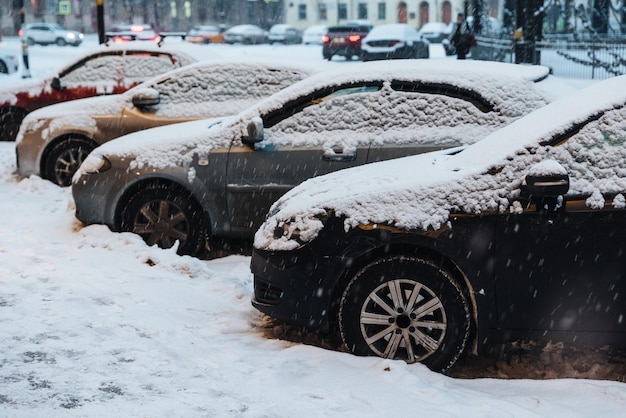In this detailed portrayal of a snowy winter day, the image features four cars parked diagonally along a snow-covered street, all facing to the left. The first car is a dark navy color, followed by a gray car, a champagne bronze car, and finally a reddish-colored car. Each vehicle is partially covered in snow, with clear visibility of the wheels and doors. The snowy sidewalk next to them shows footprints, and the curb is also shrouded in a white layer. In the blurred background, additional cars can be seen traveling with their headlights and taillights visible, along with more parked cars in front of a white building. Blurred pedestrians walk down the street and there are faint tree branches and a gated structure adorned with garland-like decorations. The predominant colors in the picturesque scene are the snowy white, the dark navy, silver, bronze, and red of the cars.